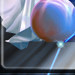This is a small, square-cropped photo featuring a medium-sized, tie-dye balloon secured at the end of a white plastic stick, which lies horizontally on a wooden table. The balloon displays a marbled effect, blending colors of blue, red, yellow, and white in a swirling pattern. To the left of the balloon lies a folded white napkin, resembling a fan, which partially rests on a gray surface and contrasts against the colorful balloon. The image is slightly challenging to decipher due to its tiny size, but the vibrant hues and arrangement of the objects stand out.